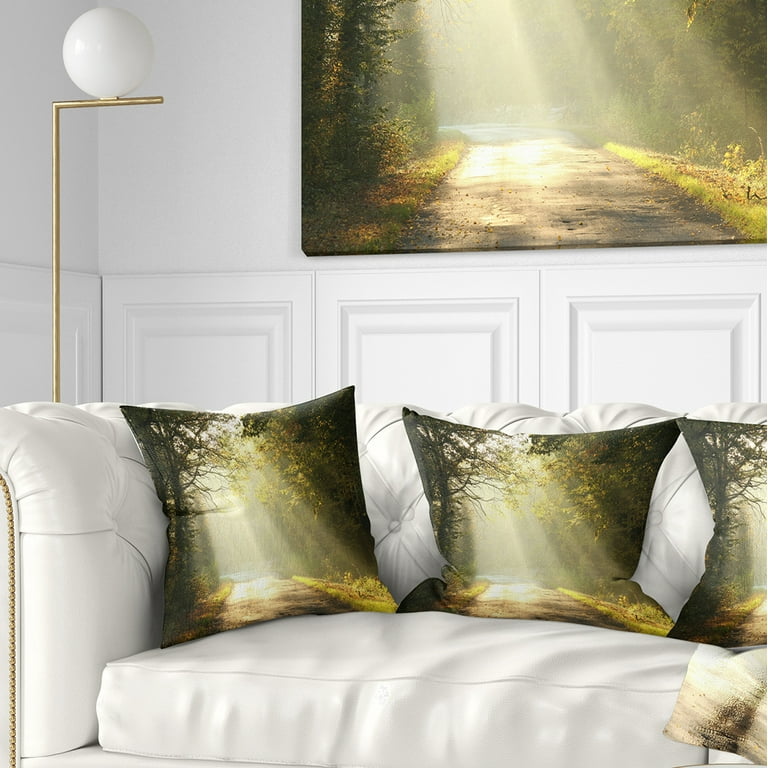In this detailed image of a living room, a white leather couch graces the center of the scene. Adorning the couch are three pillows, each displaying the same captivating image of a sunlit forest path. The middle and left pillows are fully visible, while the right one is partially obscured. The vibrant scene on the pillows reveals sunbeams piercing through trees on either side, illuminating a dirt path below. Behind the couch, the wall stands pristinely white. To the left of the couch, a stylish floor lamp with a white spherical shade and a muted gold frame adds an elegant touch. Above the couch, a large canvas mirrors the pillow design, showcasing the same serene forest path with sunlight streaming through the trees. The lower portion of the wall features paneling, accentuating the room's sophisticated charm. The couch itself, distinctly sophisticated, is detailed with gold trim along the armrests, enhancing the room's luxurious ambiance.